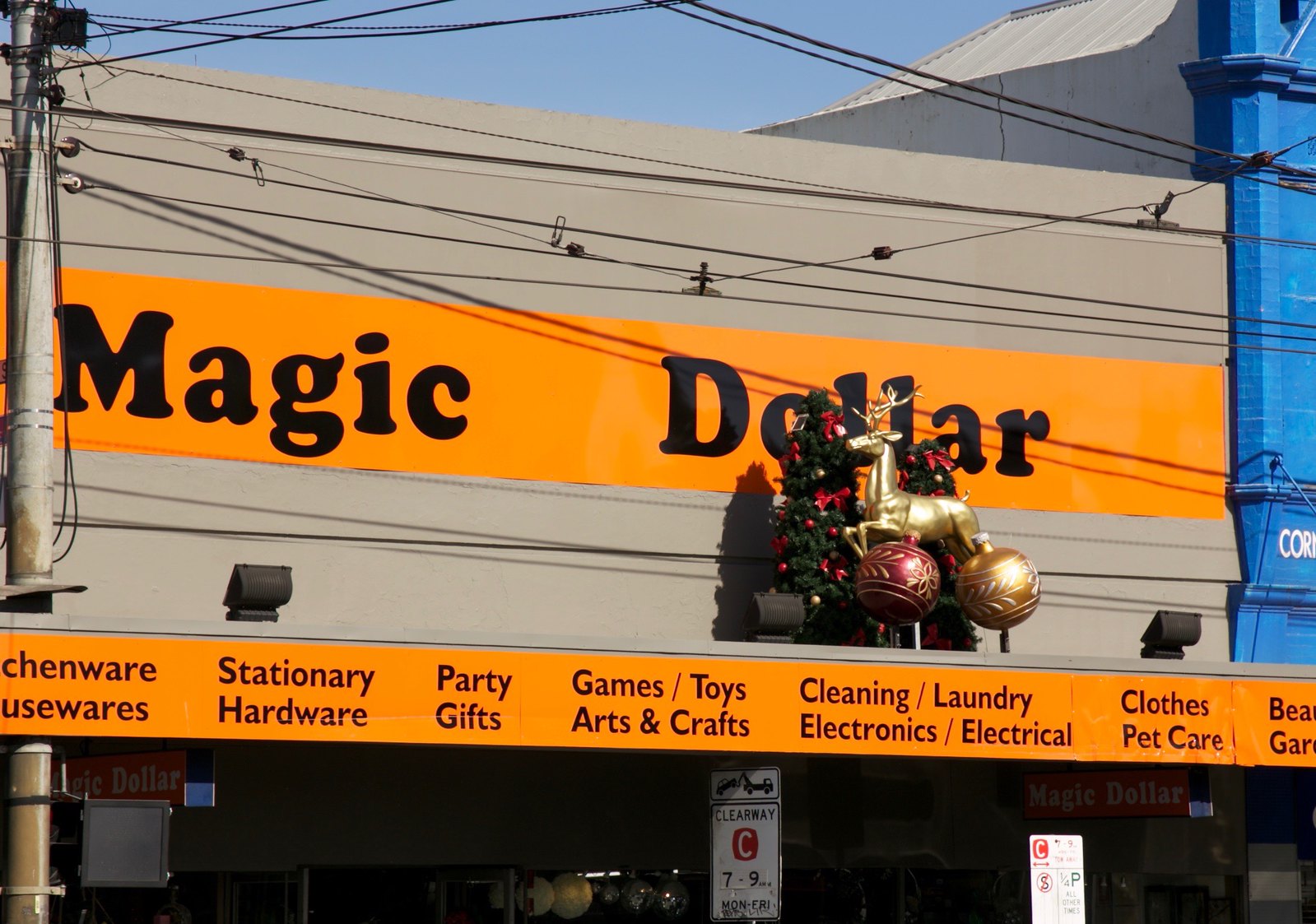The image captures a detailed view of a storefront named "Magic Dollar" on a bright, sunny day. The store occupies the majority of the frame, with just a sliver of blue sky and the tops of nearby buildings visible. An orange sign with bold black lettering spells out the store's name, and below it, a yellow banner with red font lists a wide array of items sold, including Kitchenware, Housewares, Stationery, Hardware, Party Gifts, Games, Toys, Arts and Crafts, Cleaning, Laundry, Electronics, Electrical, Clothes, Pet Care, Beauty, and more. Above the store, a tangle of power lines adds complexity to the scene. The storefront is festively decorated with artificial Christmas trees adorned with red and gold ornaments and a golden reindeer figure, creating a holiday ambiance. Several street signs and what appears to be a crosswalk are visible near the entrance, indicating a busy urban setting. The color palette includes blue, black, gray, orange, dark blue, red, and brown, adding vibrancy to the overall scene.